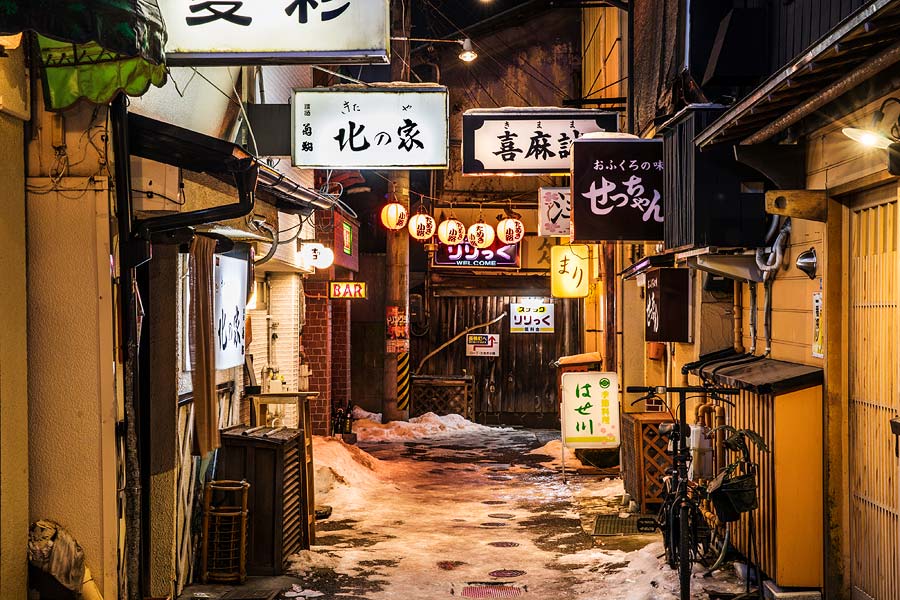In this visually captivating image, a narrow alleyway in a Japanese town stretches out under the cloak of night, adorned with a blanket of white snow and ice reflecting a soft, yellow light. The scene is segmented by cream-colored buildings on both sides, marked by numerous black and white signs emblazoned with Japanese characters. Strung between the buildings are thin strings of glowing lanterns, primarily in red and yellow, some of which are inscribed with red Japanese writing, adding vibrancy to the predominantly dark palette. In the background, a brown wooden fence and wall frame the scene, enhancing the alley's enclosed feel. A bicycle rests against the right-side building, while a yellow sign with "Bar" in red letters is prominently displayed in the middle distance above an entrance, hinting at the local nightlife. The overall composition, with its richly detailed elements and atmospheric night setting, exudes a stylistic charm that almost seems digitally rendered, blurring the lines between reality and art.